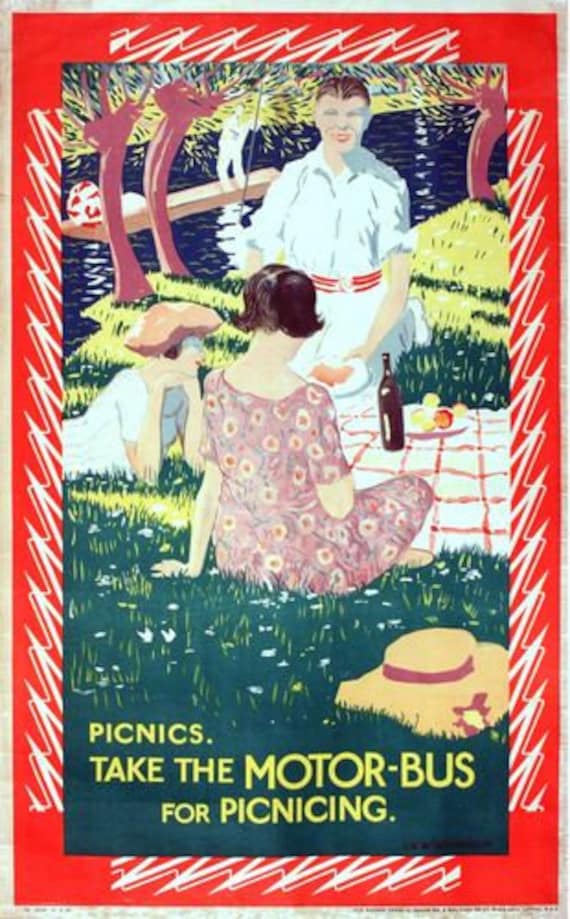This vintage illustration, evoking a nostalgic charm from the 1920s to the 1950s, serves as a promotional poster for picnicking by motor bus. The image features a quaint picnic scene bordered by a vibrant red frame adorned with jagged white stripes, reminiscent of peppermint candy. At the center is an idyllic outdoor setting where three young people—a man and two women—are enjoying a leisurely picnic on a grassy expanse sprinkled with white flowers.

In the foreground, a red and white checkered picnic blanket is spread out, adorned with a large brown glass bottle and plates, including one with what appears to be cut-up fruit or a brownish dish. The man, dressed in a white outfit resembling a sailor's uniform complete with a red belt and white short-sleeved button-up shirt, is kneeling and presenting a white plate to his companions. One woman, seated with her back to the viewer, has short brown hair and is wearing a red floral dress. The other woman, lying on her stomach with her hands resting under her chin, appears to be gazing up and smiling at the man’s gesture. She sports a brown hat.

The serene backdrop includes a gentle stream, with a lone figure navigating a gondola-style boat, and verdant trees enveloping the scene in lush greenery. In the foreground, a brown straw sun hat with a red ribbon lies casually on the grass. The illustration is completed with a promotional message in yellow font at the bottom, reading, “Picnics, take the motor bus for picnicking.”